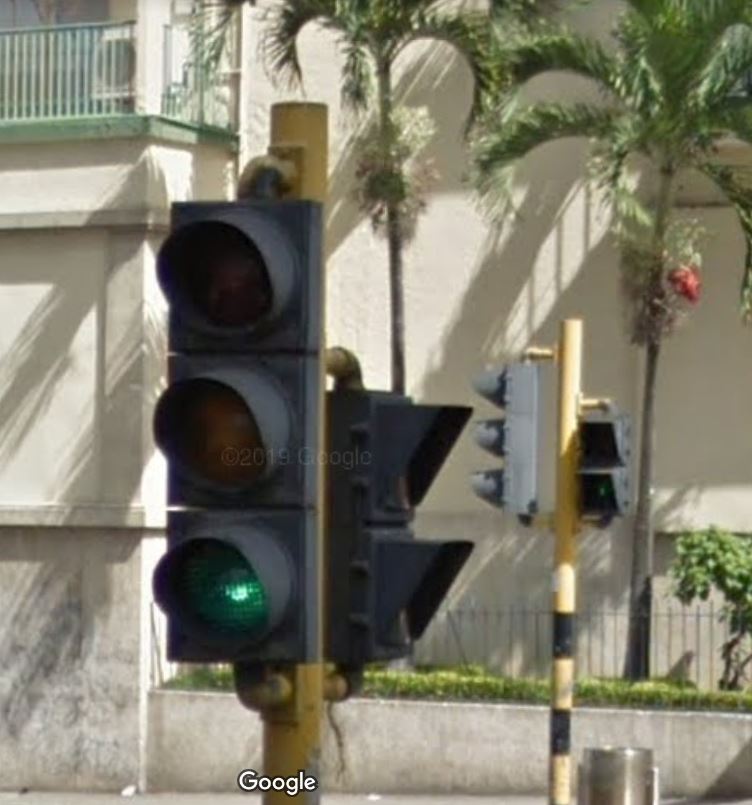The image features a close-up, cross-sectional view of a traditional traffic light with three vertical lights—red at the top, yellow in the middle, and green at the bottom—the green light is currently illuminated. The traffic light is mounted on a yellow pole with black stripes. Adjacent to this, on the right side of the image, there's another yellow pole similarly striped, featuring two square crosswalk signals. A palm tree towers in the background, with what appears to be red flowers or possibly a balloon near its top.

At the bottom center-left of the photo, there's a white "Google" logo with a black outline, indicating the image is a screenshot from Google Maps. In the bottom right-hand corner, an aluminum trash can is visible next to a small hedge and a chain-link fence, partially obscured by greenery. In the top left-hand corner, part of a tan building can be seen, featuring a balcony with a green railing and an air conditioning unit. This detailed outdoor scene captures the various elements one might find at a street intersection.